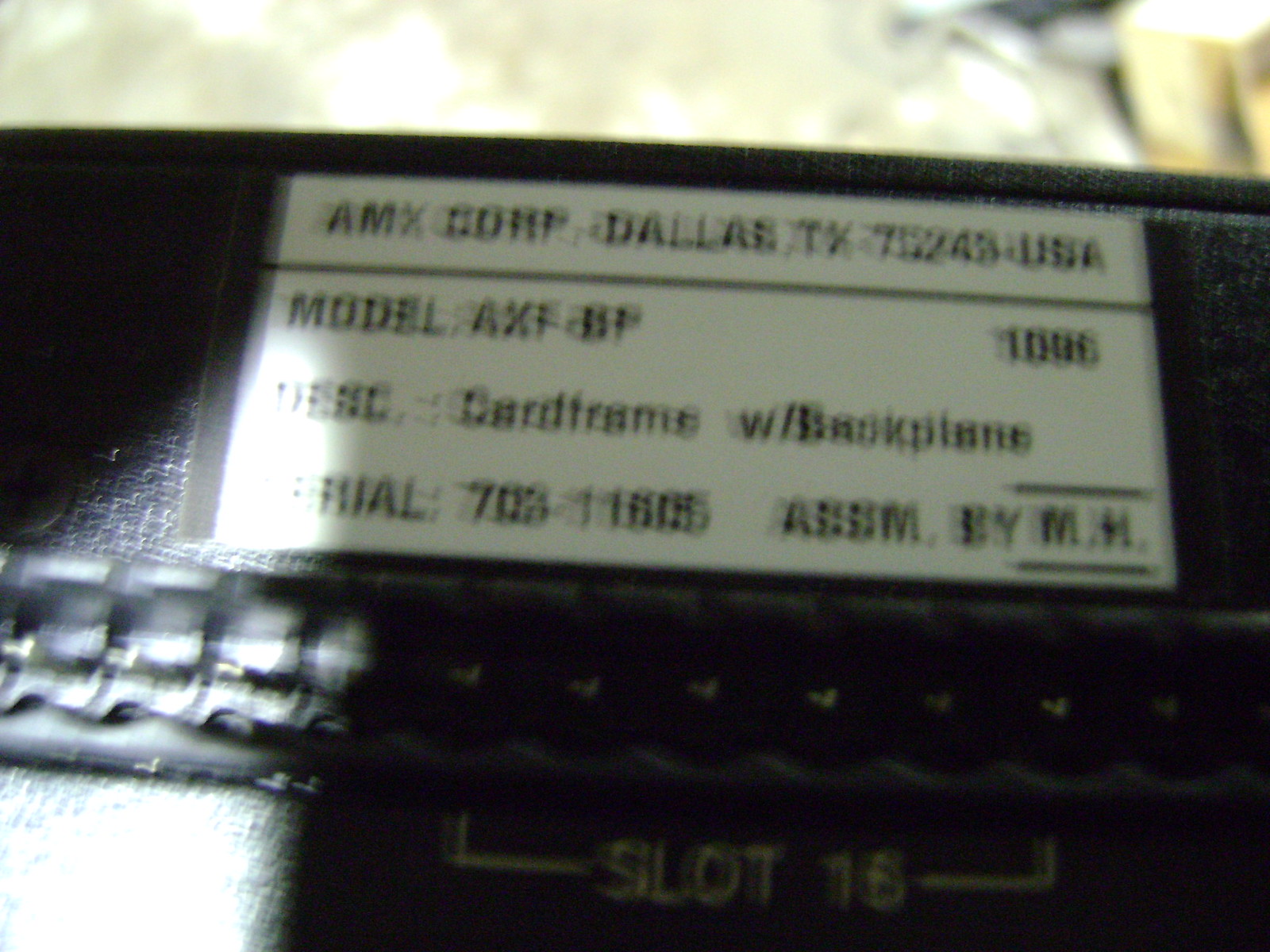The image appears to be a close-up photograph of a white tag affixed to a black item. Although the image is very blurry, certain details on the tag are discernible. The white tag includes crucial identification information such as "AMX Corp." located at "Dallas, Texas, 75243, USA." Additionally, the tag features a model number, a serial number, and the designation "slot 16." Directly above the white tag, there is a perforated strip, adding to its distinctiveness. Despite the lack of clarity in the image, these details suggest that the tag is a significant indicator of the item’s make and origin.